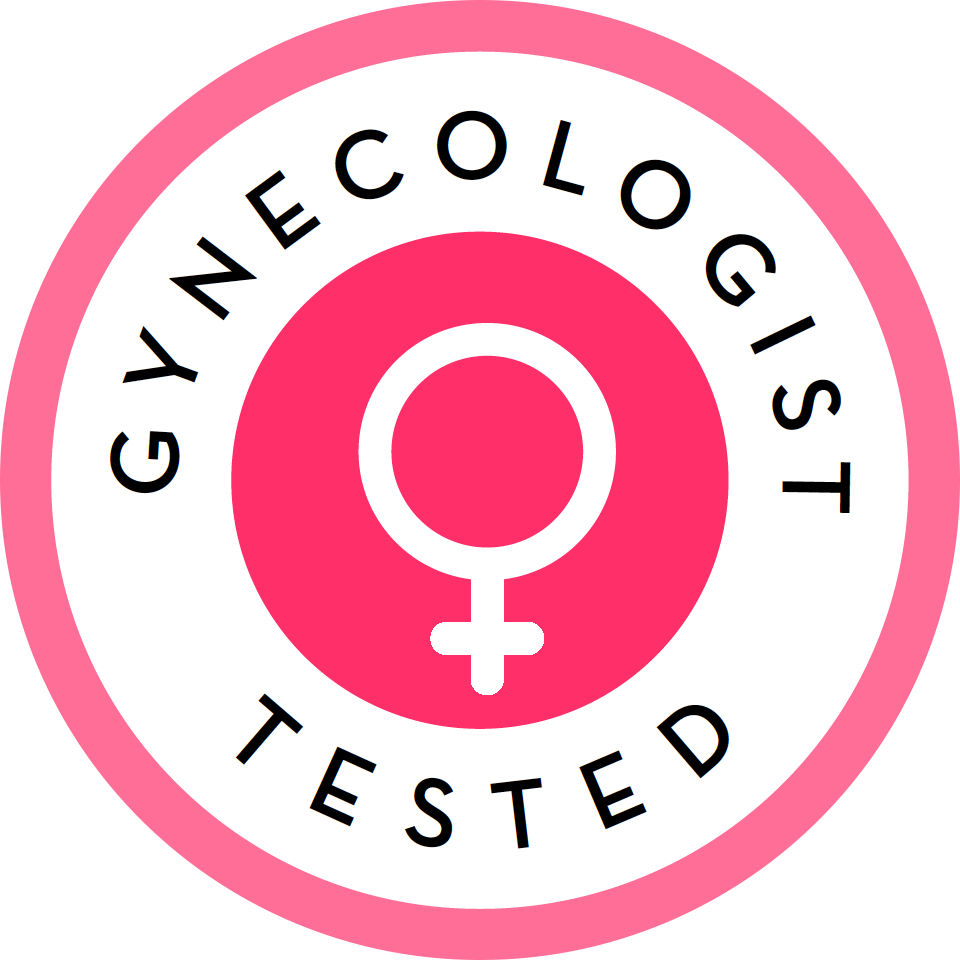The image features a circular logo with a distinct design, primarily utilizing shades of pink and white. The outermost element is a pink border encompassing a white background. Within this white section, the word "GYNECOLOGIST" is prominently printed at the top in black, all-capital letters, curving around the circle, and the word "TESTED" is displayed at the bottom in the same style. Centrally located within this design is a smaller dark pink circle, approximately half the size of the larger one. Inside this circle lies a white female gender symbol, comprised of a circle with a cross dangling beneath it. The overall appearance suggests that this logo serves as a label or seal indicating that a product is gynecologist tested and intended for women.